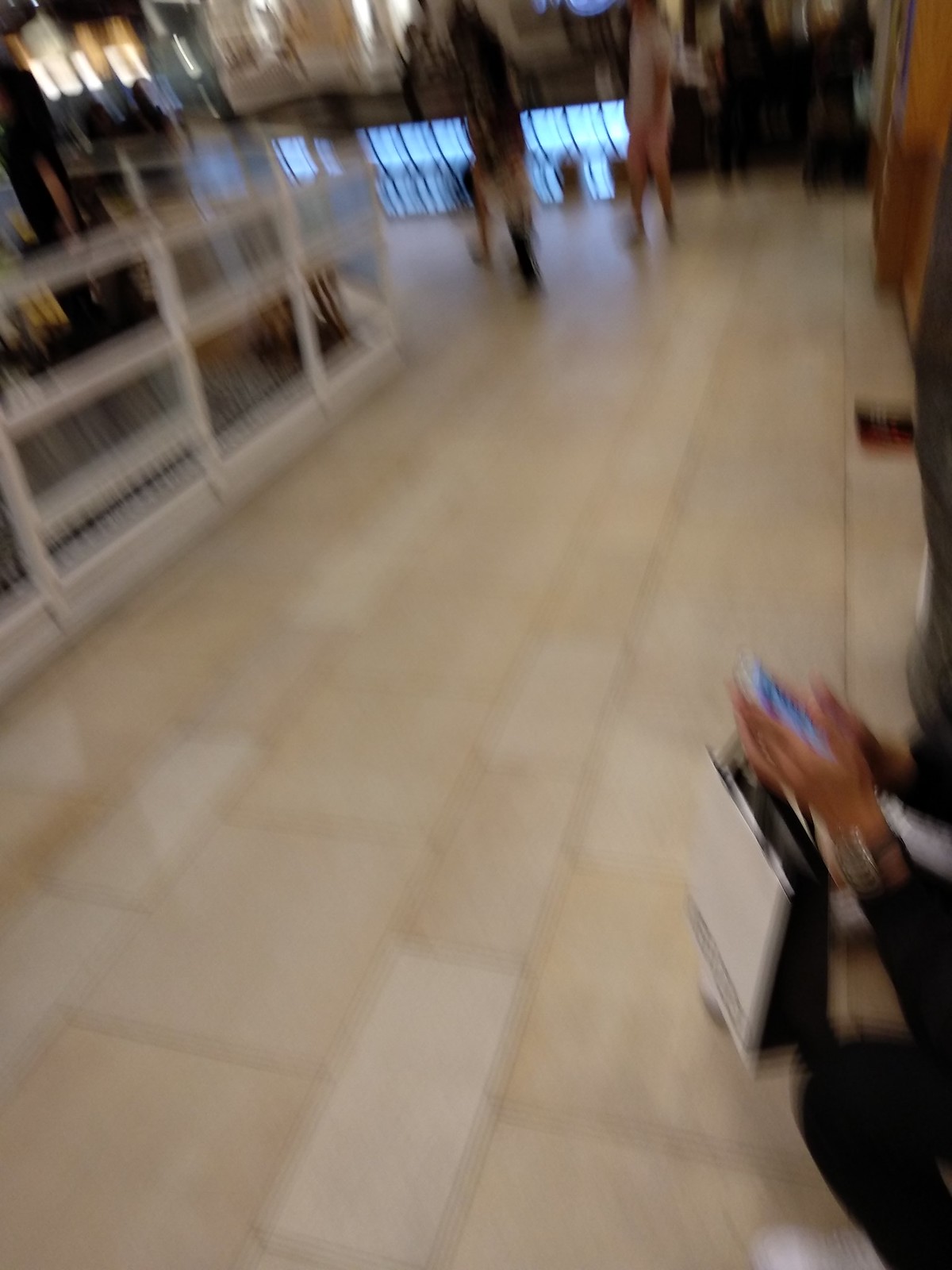This is a blurry photograph taken indoors, likely within a mall. The floor is covered in beige ceramic tiles, and on the left side of the image, a white railing can be seen. Beyond the railing and towards the background, there are two people walking: one in pink shorts and a white short-sleeve shirt, and the other in a black top. Both figures are indistinct due to the blurriness. There's noticeable lighting that suggests the presence of mall front doors on another level. In the bottom right corner, a person is crouching down, dressed in black long pants and white sneakers. They are holding a smartphone with the screen on and a small paper bag that is white with black accents and printed text. The right side of the image appears dimly lit, possibly a blocked or less illuminated walkway.